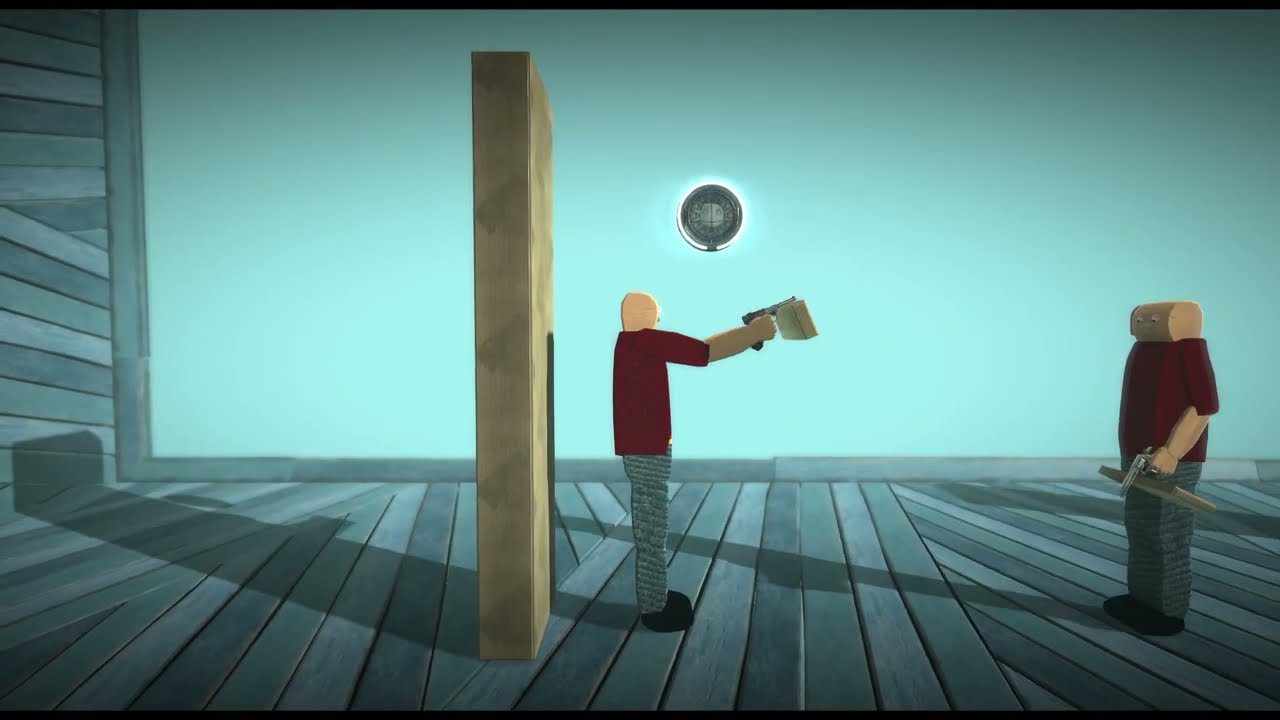The image depicts a stylized, cartoonish game interface showing two bald men with unusual head shapes engaged in a face-off, both holding pistols. The man on the left, wearing a maroon short-sleeved shirt and gray pants with black shoes, holds his gun upward in his right hand. He is positioned in front of a brown sectional wall with a light blue background behind him and stands on a gray wooden floor. His opponent, facing him on the right side of the image, has a rectangular, log-shaped head with human eyes and a slit for a mouth. He similarly wears a maroon short-sleeved shirt, gray pants, and black shoes, holding his pistol in his left hand down by his side. To the far left of the image, a gray wooden panel wall matches the flooring, creating a cohesive environment. Above the left man's head is a circle with a glowing white border, adding a distinct element to the scene.